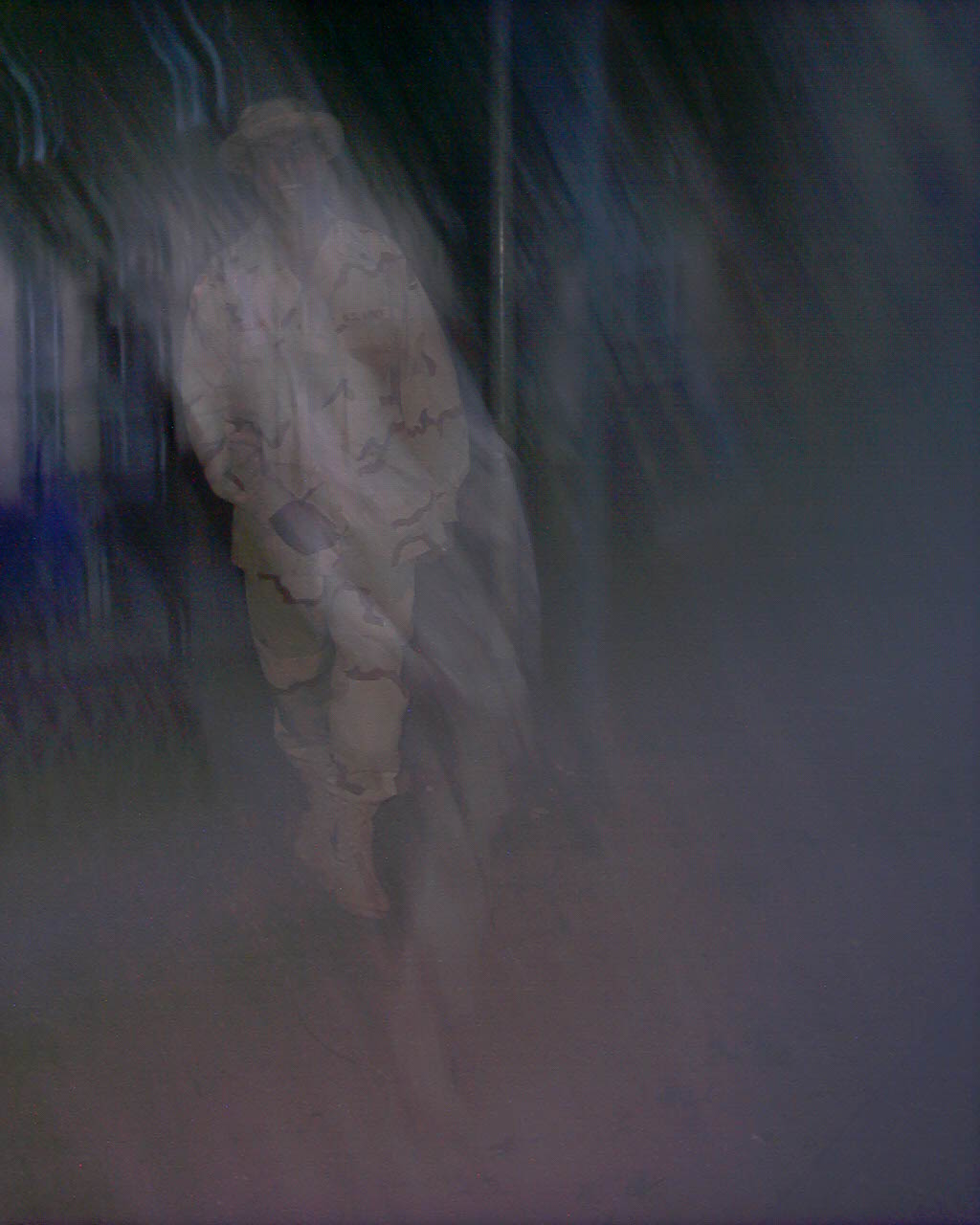The image is a very dark, grayscale photograph, almost entirely black with indistinct, ghostly shapes. The primary form is a blurred figure, possibly a person or a creature, adding to its mysterious quality. The ambiguity makes it look ghost-like, with four protrusions that resemble tentacles, suggesting the alternate possibility of it being a sea creature like a squid. However, another interpretation suggests it could be a moving figure, possibly a man in a camouflage outfit, complete with a jacket, pants, boots, and a hat. Despite the dark and blurry nature, some details are visible: 
   - Rounded rectangular patterns with one appearing almost filled in blue.
   - A central object that could be a pipe or a post.
   - Potential background elements like blurry houses with white shutters and a patch of grass.
The overall darkness and ghostly appearance make the exact subject almost impossible to distinguish.